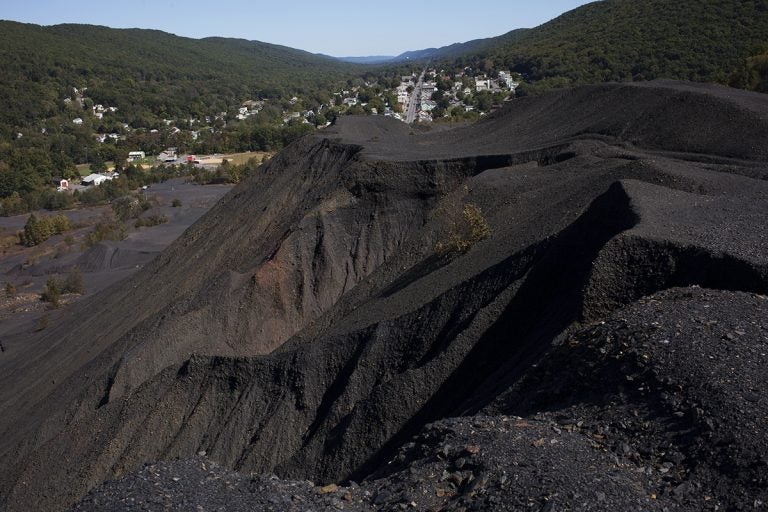This daytime photograph captures a diverse landscape composed of dramatic geological and botanical elements. The backdrop is a clear blue sky with a few distant buildings nestled amid lush, thick forests that cover the rolling hills on both the left and right sides of the image. The primary focus of the image is a striking rock formation that dominates the foreground. This formation appears almost black, with charcoal gray and dark brown hues, suggesting it could be composed of ancient cooling lava or coal. The steep, jagged slopes of the formation are largely devoid of plant life, save for one small, scraggly bush clinging to the dark soil. Behind this rocky expanse lies a town engulfed in greenery, with copious trees and some scattered fields. The town is connected by a main road and features numerous buildings, blending into the wooded surroundings. Further into the distance, beyond the black hills and the town, the landscape transitions into more low-lying hills, completing this scenic, mountainous vista.